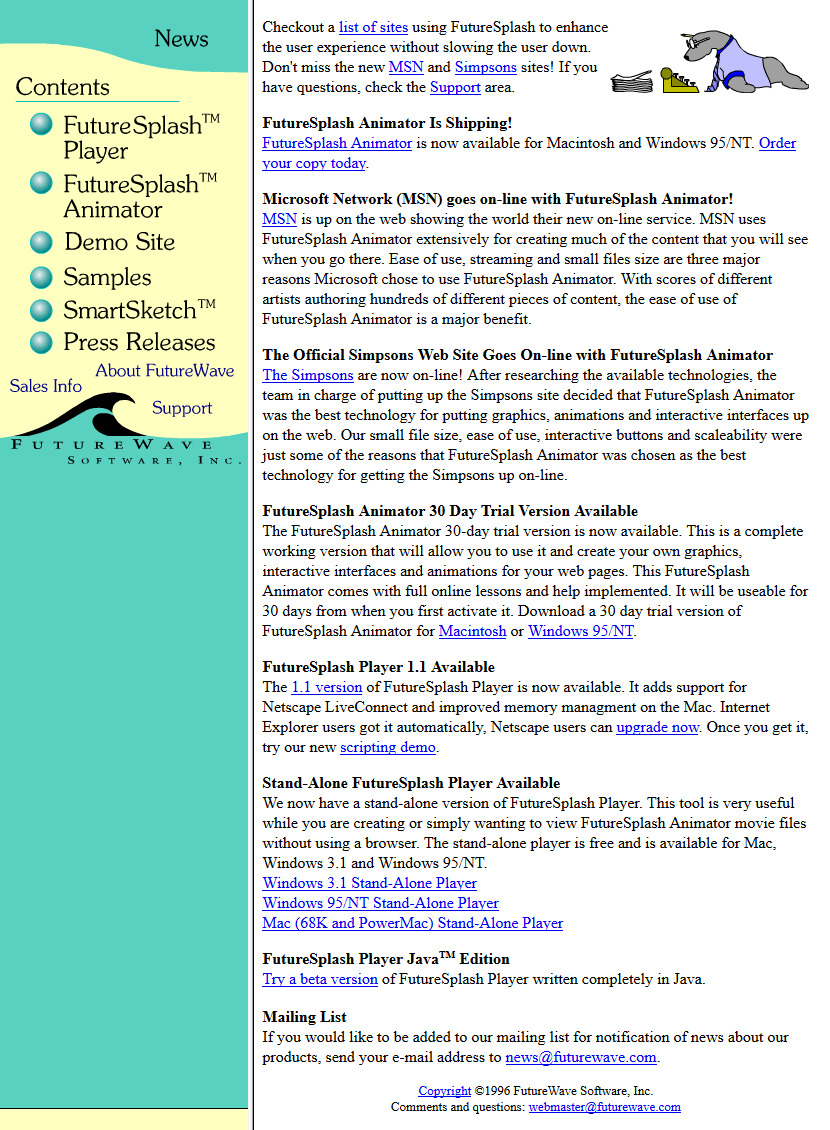The image portrays a nostalgic webpage or document page, reminiscent of the mid-90s era. The layout is split into two distinct sections: a left-hand navigation pane and a right-hand content display area. 

On the left, a turquoise-colored panel features a structured list of clickable items. The list begins with "News" and "Contents," followed by options such as "Future Splash Player," "Future Splash Player Animator," "Demo Site," "Samples," "Smart Sketch," and "Press Releases." Below this list, the name "Future Wave Software, Inc." is prominently displayed.

The right side of the image serves as the main content area, displaying text against a white background. The text promotes the "Future Splash" suite of products, highlighting how they enhance user experience without compromising performance. It specifically mentions notable sites like Emerson and Simpson utilizing Future Splash. Information about product support and the announcement that "Future Splash Animator" is now available for both Macintosh and Windows 95 NT is included, urging users to order their copy. Additionally, details about various updates and features of the Future Splash products are provided.

At the bottom of the page, there is a copyright notice stating "© 1996 Future Wave Software," and contact information for the webmaster is given as "webmaster@futurewave.com."

Overall, the page showcases a typical 90s design with a left-sided navigation pane and a main body of text focused on product updates and company information.